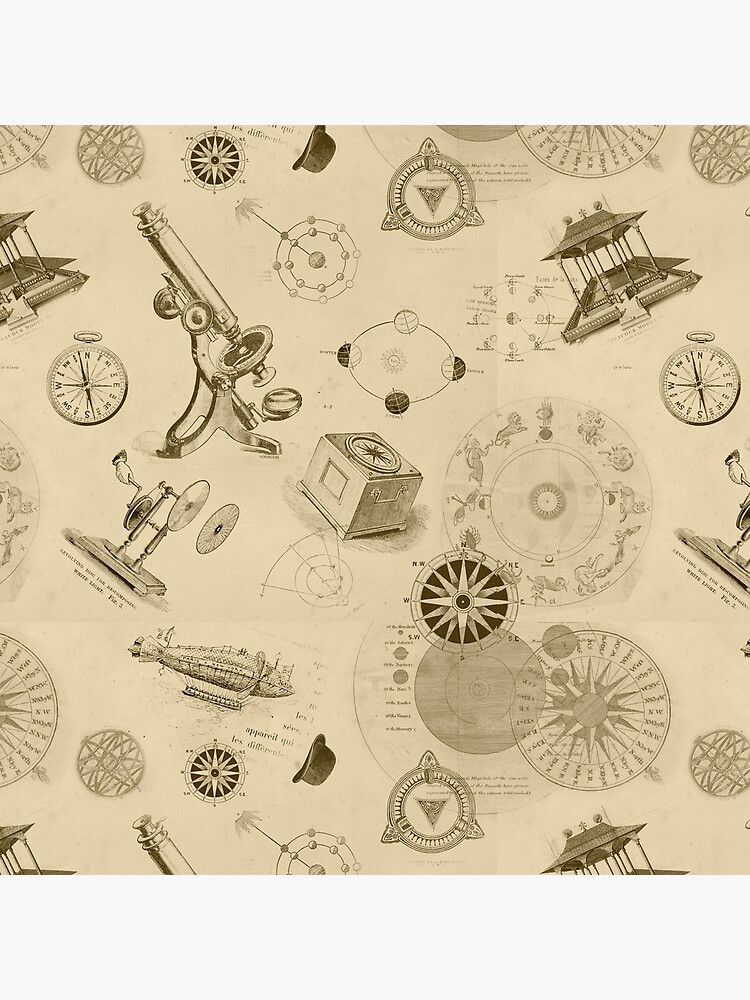The image is a vintage, sepia-toned drawing depicting an eclectic array of scientific instruments and inventions. Dominating the top left is a detailed illustration of a microscope, emblematic of scientific exploration. Directly beneath it, an archaic device with cranks and wheels hints at early mechanical engineering. Adjacent to this, a fantastical depiction of what could either be a submarine or an airship adds an element of adventure and invention.

Scattered throughout the composition are several circular devices, including dials, compasses, and perhaps even stopwatches, adding to the navigational theme. The top right corner features an architectural structure resembling a pagoda or a gazebo, lending an exotic or astronomical flair to the drawing. At the very top center, an upside-down bowler hat adds a whimsical touch, perhaps symbolizing the era or the thinkers of the time.

Additional elements such as telescopes, solar system illustrations, zodiac signs, and possibly a vintage airplane, as well as various logos and directional pointers, enrich the composition. The background is an off-white, aged paper that enhances the antique feel. Despite the chaotic and haphazard arrangement of these black, white, and gray illustrations, each item contributes to a broader theme of scientific curiosity and invention.